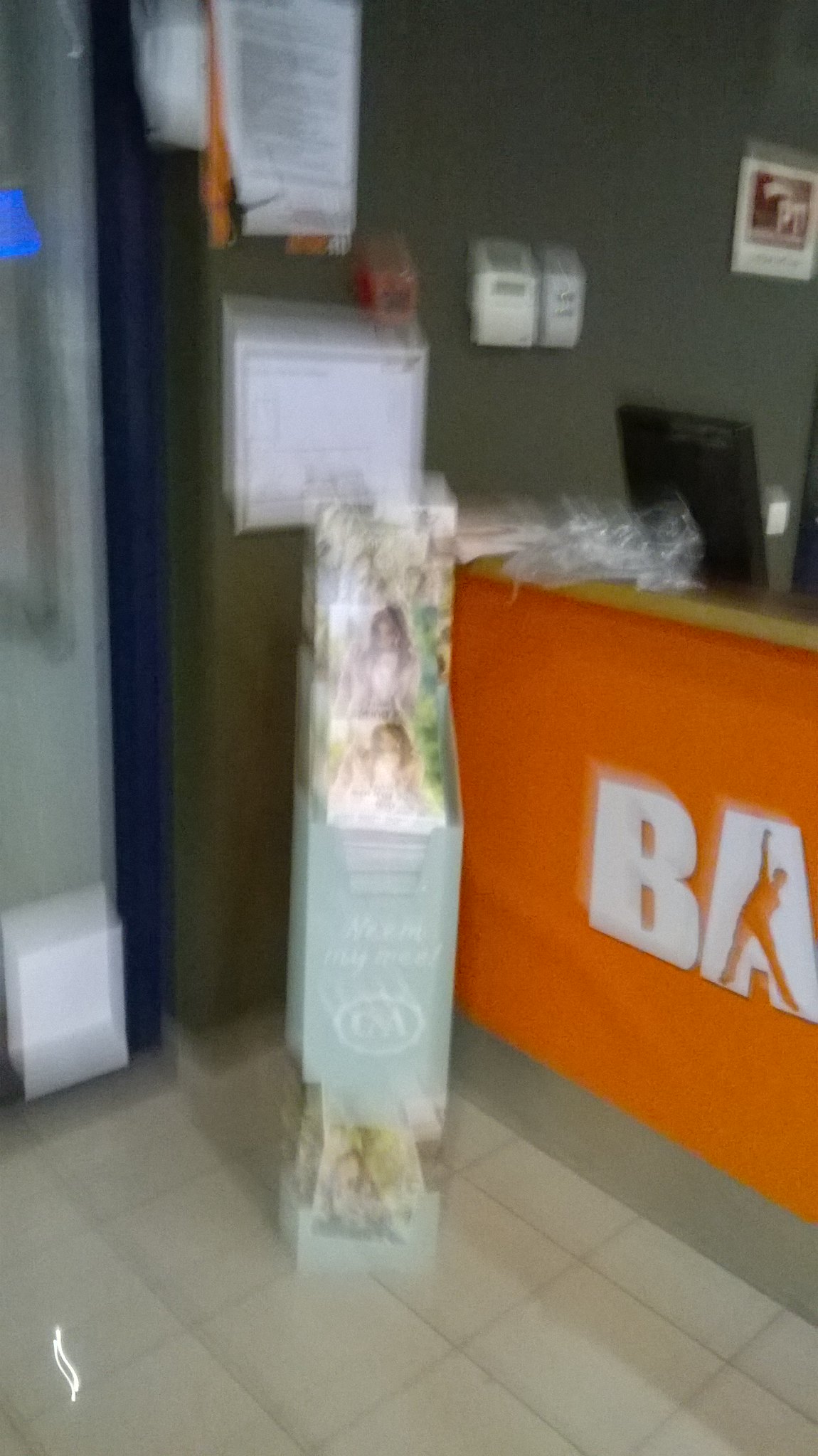The image captures the interior of a professional office setting, as seen through a vertically rectangular frame. The scene is quite blurry, making some details hard to discern clearly. In the background, a dark green wall is visible, adorned with various pieces of signage and a thermostat situated prominently. From the center of the frame, a tan countertop tilts downward towards the right center of the image. Draped over the front of this countertop is a large orange banner, displaying the partially visible letters "BA." To the left of the countertop, a narrow, vertically rectangular display stands, presumably holding an assortment of pamphlets. Despite the overall blurriness, the structured arrangement and elements within the office hint at a professional work environment.